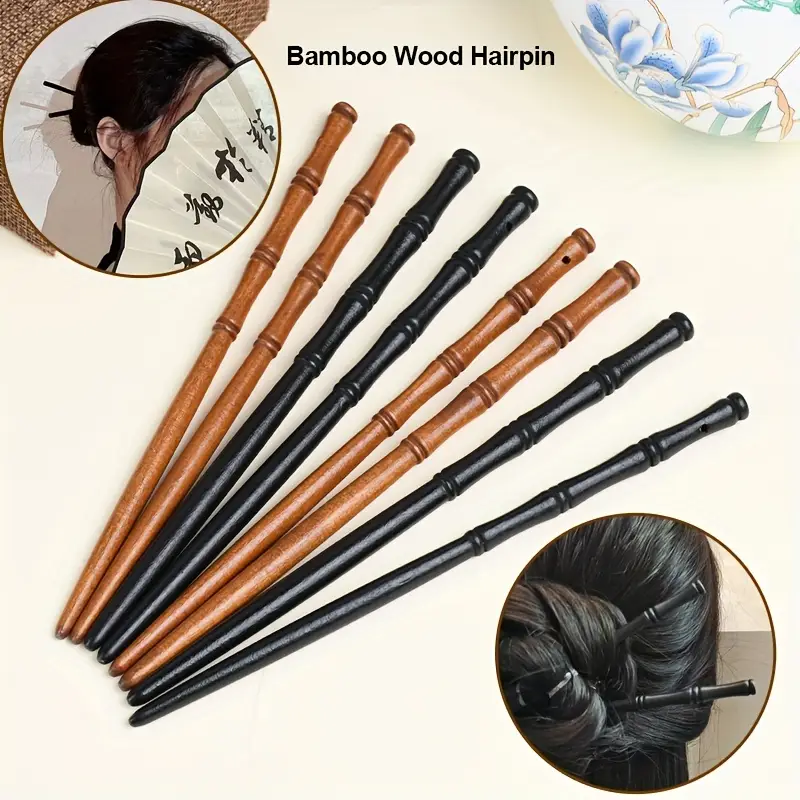The image showcases a product display for bamboo wood hairpins against a cream-colored background. Centered prominently are four pairs of these hairpins, arranged meticulously in the middle. Starting from the left, the first two pairs are a medium-toned brown, followed by a pair of very dark black hairpins, another pair in the medium-toned brown with one featuring a distinguishable black spot near the top, and finally, another pair in the very dark black. Notably, the hairpins are narrower and rounded at the bottom but fan out towards the top. 

In the upper left corner, there's a circular inset photo of a woman’s head viewed from the back. She is holding a white fan with what appears to be Chinese or Japanese characters which obscures her face. Her black hair is elegantly pinned up with white sticks protruding stylishly. In the bottom right corner, another circular photo provides a closer view of the same woman’s bun, giving a detailed look at the black hairpins holding her hair in place. In the upper right-hand side of the image, there is a small cup adorned with a blue flower. At the very top, the text "Bamboo Wood Hairpin" is inscribed in black letters, tying the whole visual presentation together.